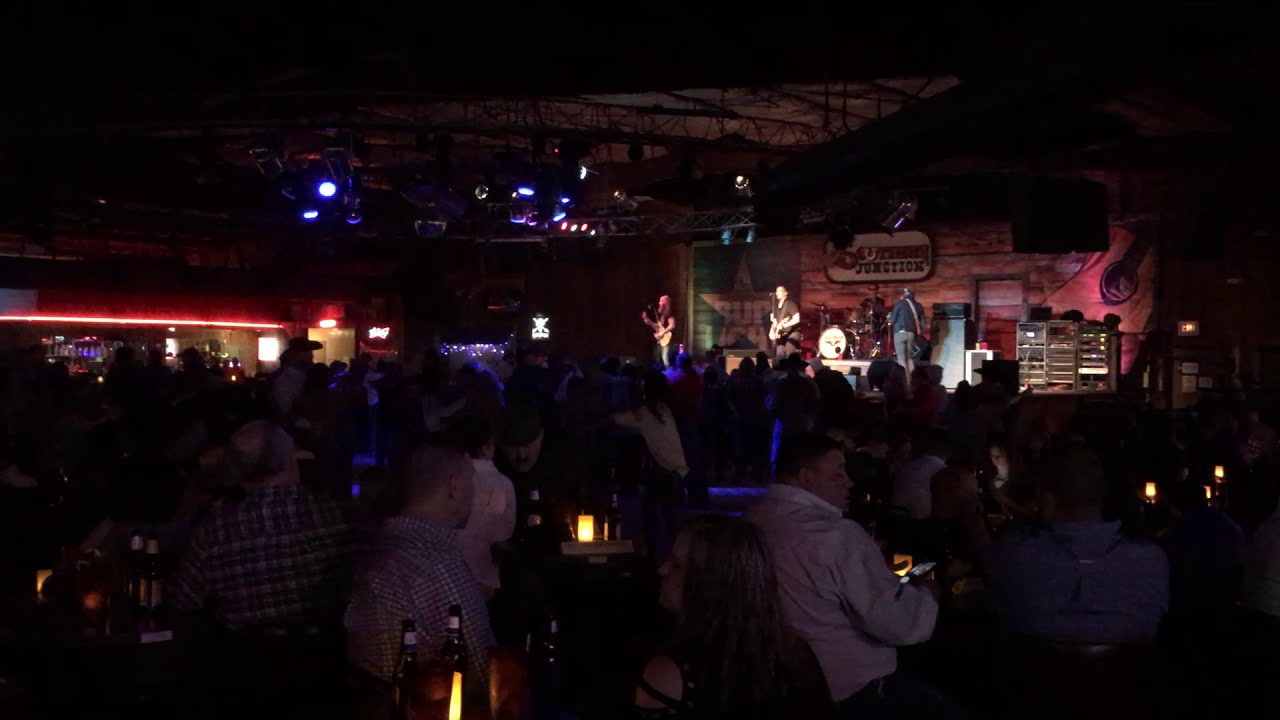The image depicts a dimly lit bar and concert venue, featuring a wooden stage adorned with the Texas flag and a painted guitar. A band is performing; two guitarists, a drummer, and a banjo player are visible against a backdrop sign that reads "Junction" in red and black letters. The cozy room is filled with patrons, around fifty, seated at round tables softly illuminated by candlelight, each table adorned with glass beer bottles. Overhead, blue and purple lights cast an ambient glow. To the middle left, a bar with a long, red glowing strip at the top is visible. The overall atmosphere suggests a lively yet intimate concert setting within a rustic bar.